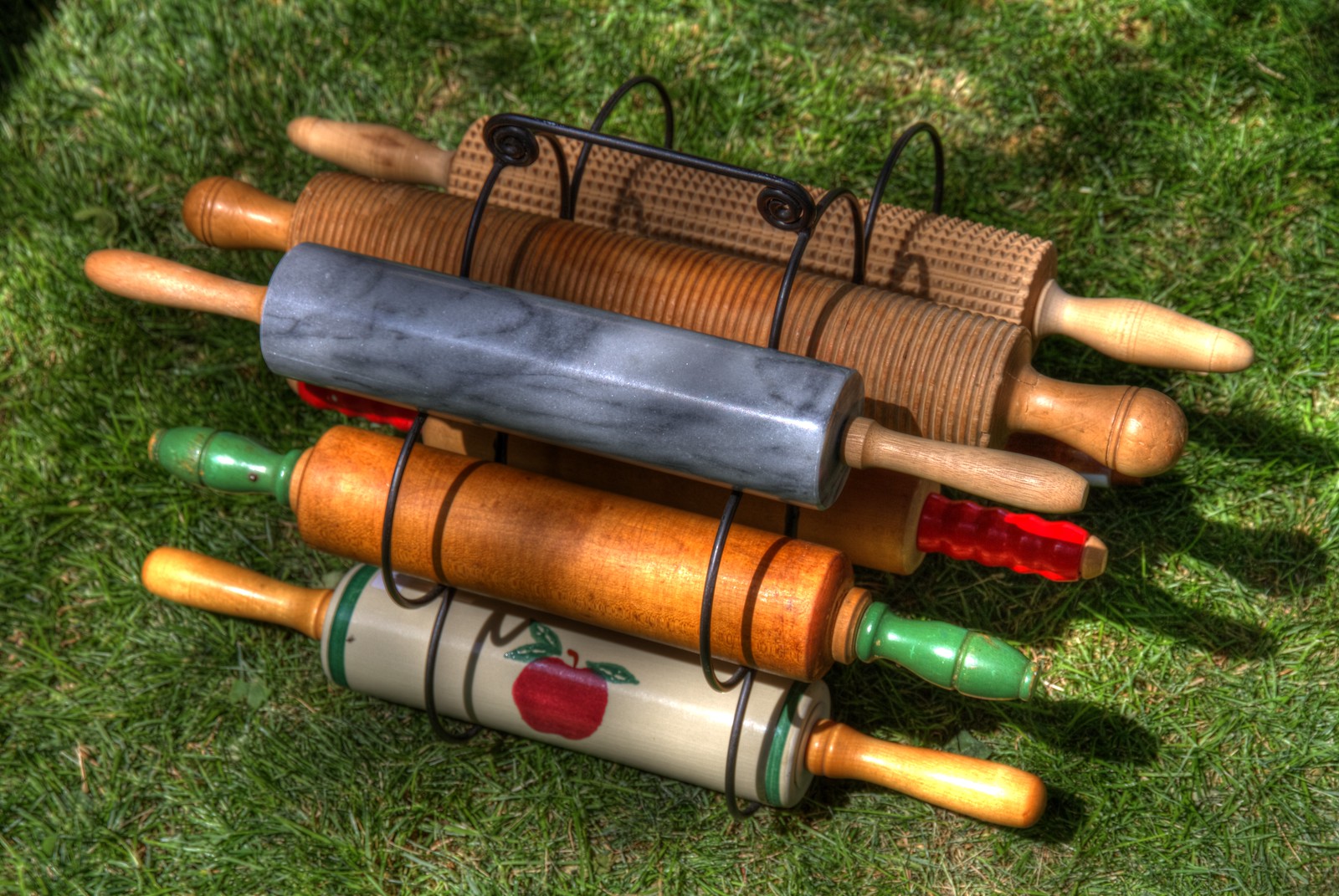The photograph captures an assortment of six distinct rolling pins arranged in a black metal wire holder, placed on a green grassy lawn. Each rolling pin showcases unique features and materials. At the bottom, a rolling pin with a white central section features green stripes at the ends and a bold red apple with green leaves painted in the middle. This one sports orange wooden handles. Above it sits a rolling pin made of darker orangey wood, adorned with intricately carved dark green handles. The next one appears to be crafted from marble, exhibiting blue and black marbling and complemented by longer, softer, beige wooden handles. In the central back, there's a wooden rolling pin with bright red ribbed handles. Another rolling pin, also wooden, features lined textures across its middle section and has thicker, shorter handles. Finally, the one at the back has a series of small spikes on its central wooden section and is completed with long, light wood handles. There might be a seventh pin barely visible, peeking out from behind the others, adding to the quaint and diverse collection displayed in this outdoor setting.